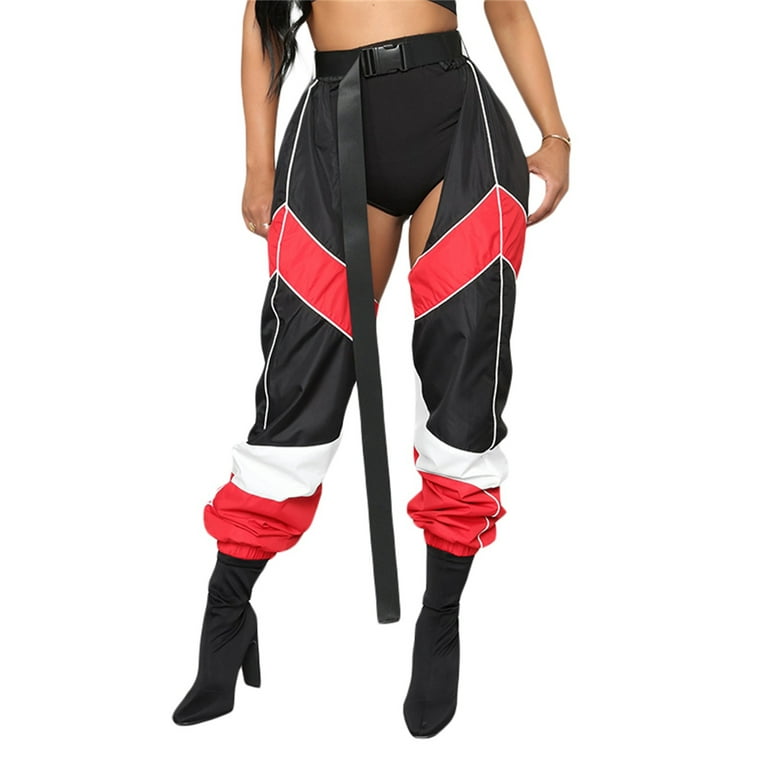This product image, shot against a white background, features a woman from the midriff down, emphasizing a pair of distinctive parachute-style pants. The woman, with long black hair partially visible in the upper left corner, is wearing a black fabric belt with a plastic buckle, which extends nearly to her high-heeled black boots. She also sports a silver bracelet on her left wrist. The pants are an eye-catching design primarily in black, adorned with a red chevron stripe at the thighs and white piping outlining the red. Below the knee, there is another white stripe followed by a red band near the ankles. Notably, the pants are open at the crotch area, revealing her black underwear and the inner sides of her thighs. The pants appear to be made from a material similar to that used in parachutes, contributing to their unique, edgy aesthetic.